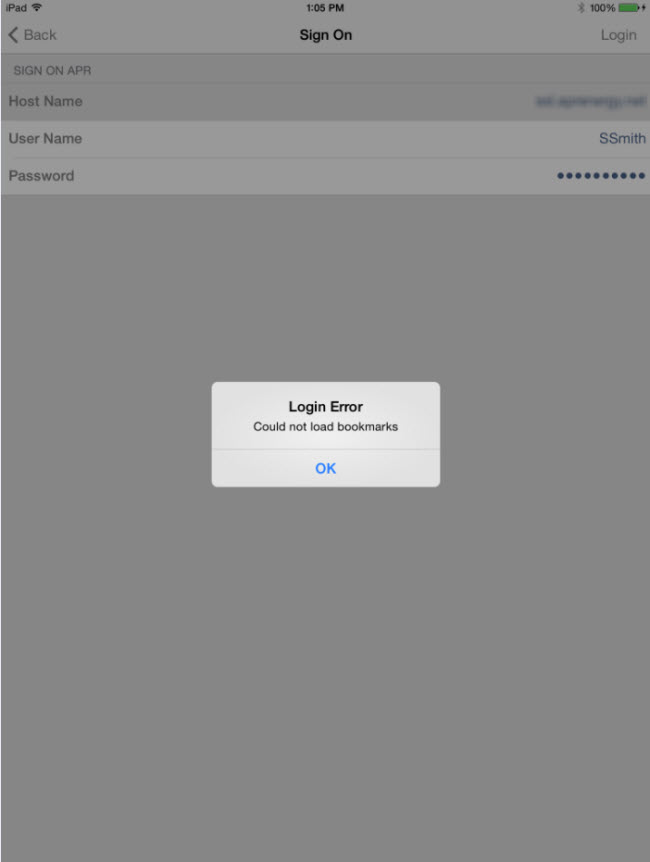The image depicts a login interface on a website, displaying the time as either 1:09 PM or 1:05 PM. The central focus is a prominent "Sign On" heading in large black letters. The battery status is shown at 100%. On the right side of the screen, the words "Log In" are visible.

The interface includes several gray bars, each serving different purposes. The first bar, titled "Host Name," is dark gray. Below it is a lighter gray bar for "Username," where "SS Smith" is displayed on the right side. Another gray bar is designated for "Password," with black dots concealing the inputted characters for security.

A white box in the center highlights a "Log In Error" message, stating "Could not load bookmarks." Below this message is a blue "OK" button. The entire section with the error message is surrounded by a dark gray background, matching the color of the upper gray bars.

No company name or branding is present, indicating this is a generic sign-on page where the user has encountered an issue with loading their bookmarks. The system does not provide any instructions for resolving the error, merely suggesting they may need to press "OK" and try again.